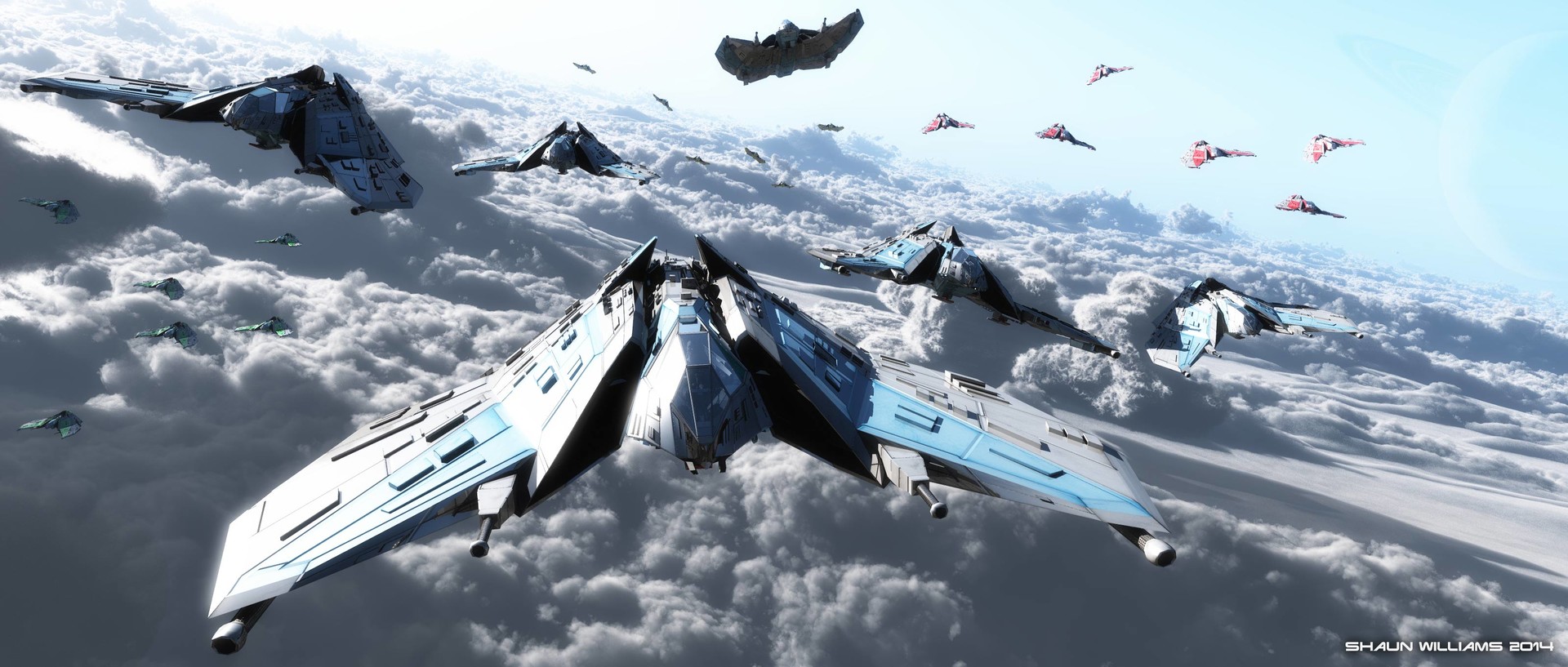The digital image by Sean Williams from 2014 features a highly detailed, 3D-rendered sci-fi aerial scene. The focal point is a squadron of futuristic spacecraft resembling space-age fighter jets, equipped with blasters and streamlined wings integrated smoothly into their bodies. The foreground showcases at least five large jet-like ships with prominent blue accents on their wings, while numerous smaller, similarly colored ships trail behind. These vessels are positioned above a sea of swirling clouds, casting shadows upon them.

In the distance, a fleet of smaller, red-accented ships appears, perhaps indicating a rival faction in this speculative setting. The scene exudes a dynamic tension, intensified by the contrasting colors and the strategic formation of the vehicles. Overhead, the sky transitions to a lighter blue, and a soft sunlight permeates, casting a surreal glow over the entire tableau. Moreover, on the right edge of the scene, a majestic planet with a visible ring structure—reminiscent of Saturn but tinged blue—adds an extra layer of depth and wonder to the composition.

This meticulously crafted work, signed by Sean Williams in small white text on the bottom left, seamlessly blends elements reminiscent of gaming and science fiction, invoking a visual narrative akin to what might be found in franchises like Halo or Star Wars.